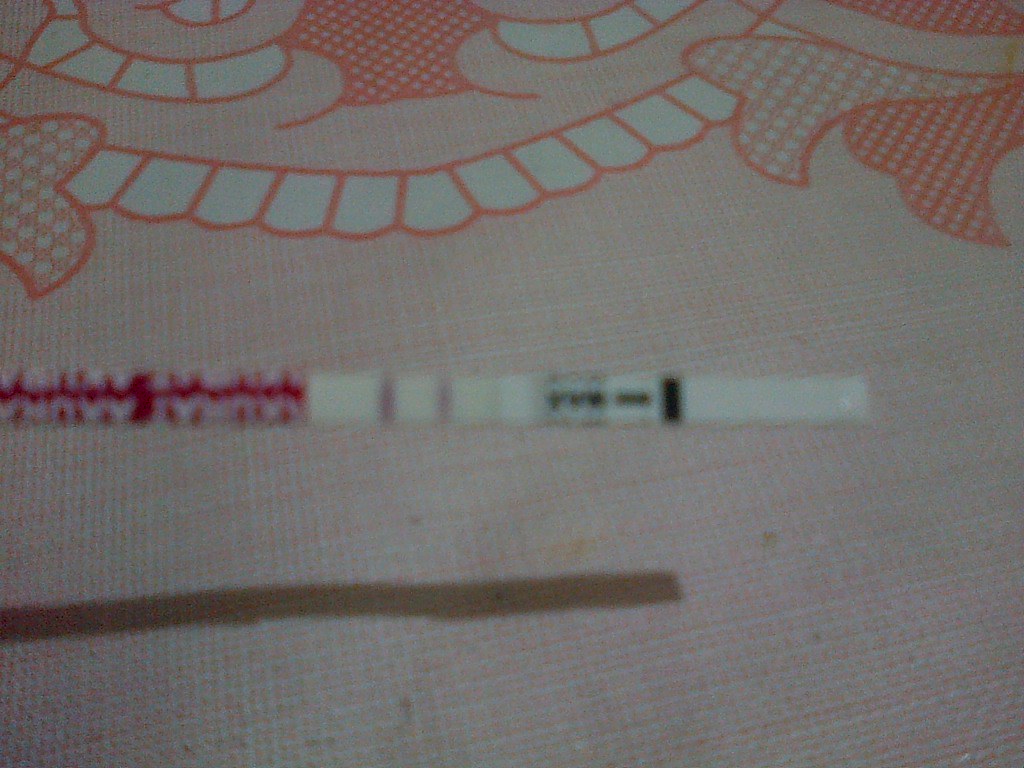The image depicts a somewhat out of focus, intricately woven piece of cloth. In the foreground, the fabric features a tightly woven pattern in vibrant pink and white. Additionally, a shadow covers the majority of the left three-quarters of the image. Above this section, the color shifts to red and white on the left, transitioning to white in the middle, then changing to black and white for a brief section, before becoming predominantly white again about 80% across horizontally. 

This woven piece is not very wide, adding a compact charm to its design. Above the blend of colors, there's a distinct pattern resembling stylized teeth, rendered in white and red. These “teeth” arch upwards, creating a smile-like curve, and are flanked by pink flowers with white dots on each side, adding a decorative touch. Below one of the pink flowers, a red flower with horizontal white stripes introduces another colorful element. 

Above the teeth pattern, more shapes are delineated, resembling additional teeth, separated by what could be interpreted as a nose featuring the same red and white patterned design seen in the flower on the right. On each side of this 'nose' are outlined shapes that enhance the detail of the piece. In the upper right corner, there is a shape that intriguingly resembles an eye, completing the complex and detailed woven artwork.